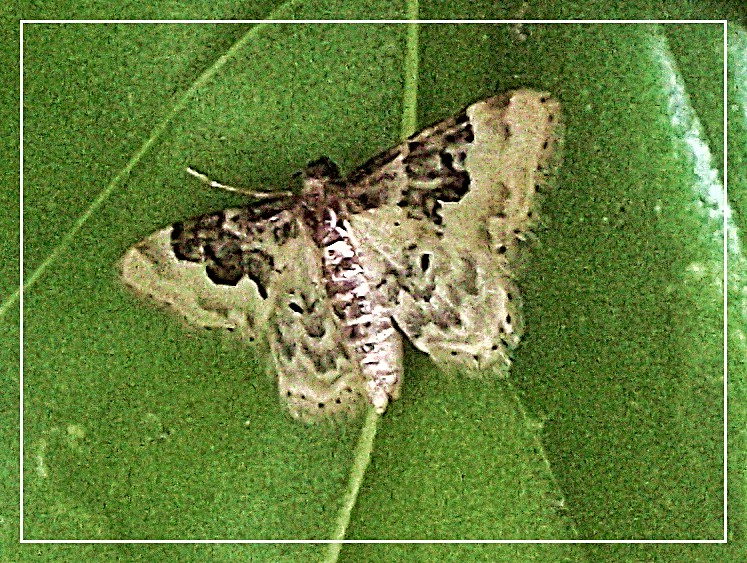This detailed photograph, oriented in landscape, showcases a beige and brown moth resting on a dark green leaf. The moth, with its elliptical body featuring horizontal bands of dark brown and cream colors, is angled slightly, with its top right wing pointing towards the top right corner and its left wing extending towards the middle left of the image. The moth's wings exhibit a speckled pattern of brown, white, and light brown, while a single white antenna protrudes from the top left of its head. The leaf beneath the moth is dark green and distinctly veined, with the primary veins being light green and one particularly lighter white vein in the upper right corner. The leaf surface presents a speckled finish transitioning from dark green to lighter green. The entire still life exudes photographic realism, capturing the intricate details of both the moth and the leaf meticulously. There is a white inset rule near the border, emphasizing the precision of the composition.